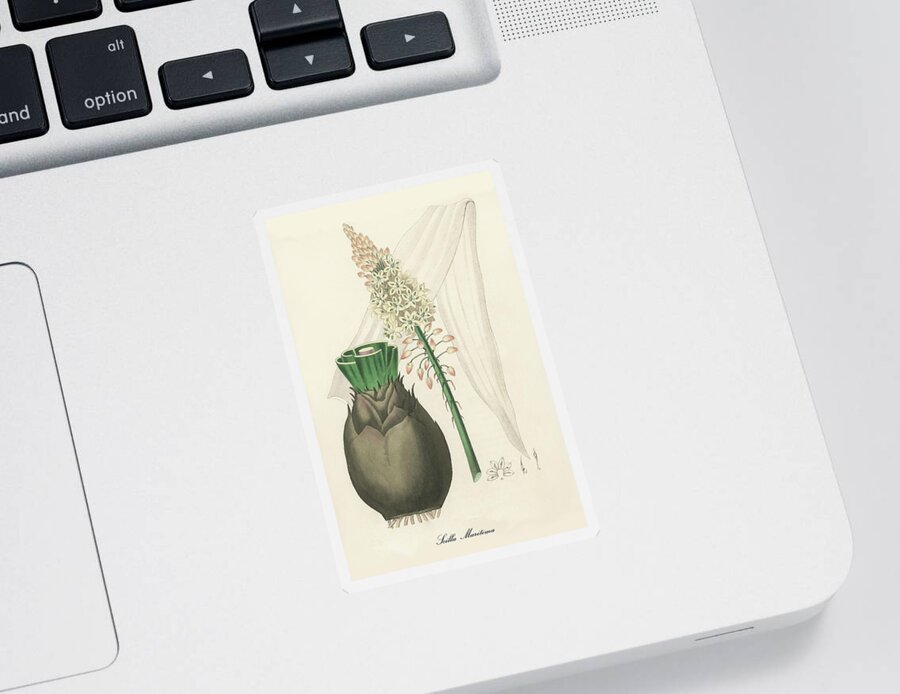This image depicts a white laptop with a black keyboard, showcasing the Alt, Option, and directional keys, alongside the trackpad on the left side. In the lower right corner of the keyboard, a cream-colored postcard or sticker is attached. This sticker features a detailed, multi-element design. Central to the sticker is a vase-like illustration or an odd-looking unopened flower, characterized by a dark base and green shoots, with a yellow center that hints at potential blooming. Beside it, there’s a fancier flower with a red base, small buds, and intricate petals. Complementing these floral elements is a see-through, fine scarf or cloth design that drapes behind the flowers and downwards, resembling a delicate, sheer curtain blowing in the breeze. Small, cursive text is present on the sticker, likely inscribed with a name, though it is too small to be legible.